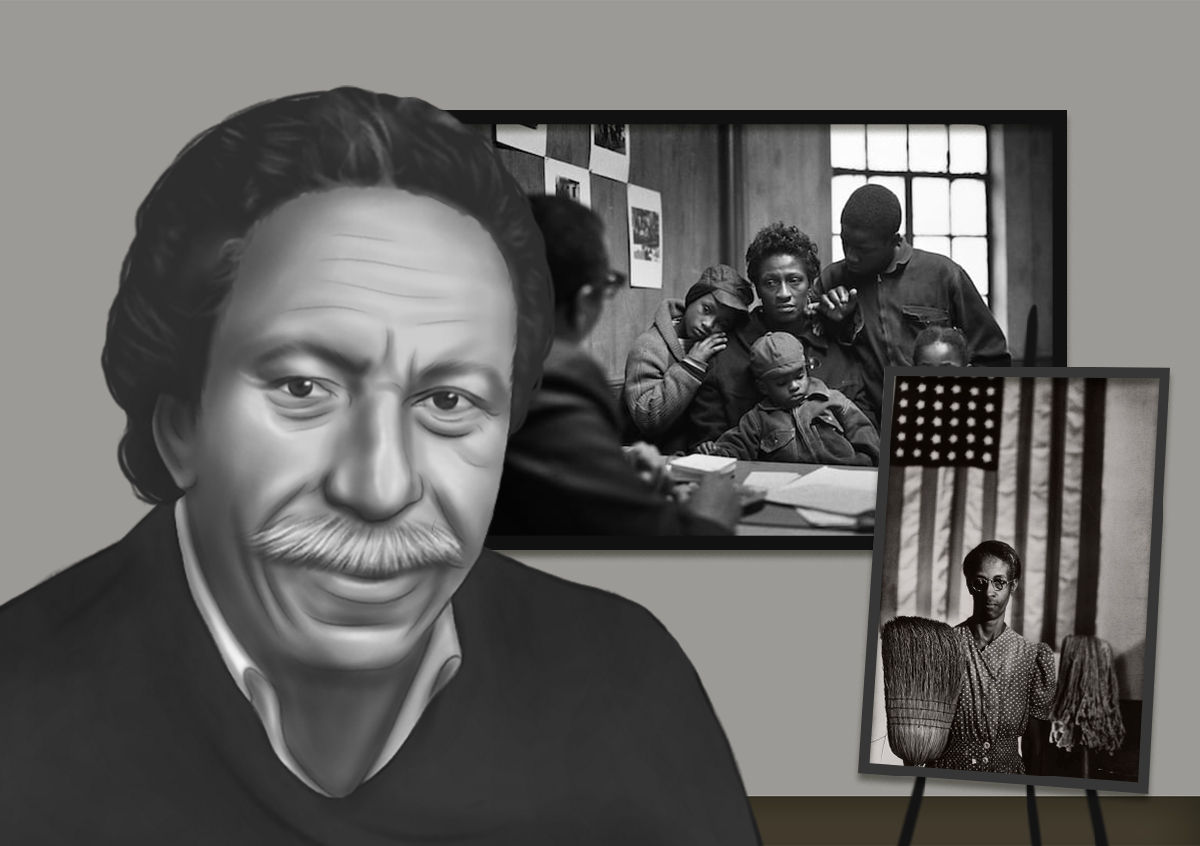In the foreground of this detailed black and white drawing, there is an older African American man with a wrinkled face and a white mustache. His hair is slicked back, and he wears a dark shirt—possibly black or dark blue—with a white collar underneath. He has an expression that suggests seriousness. Behind him, two photographs are visible. 

The first photograph depicts a seemingly stressed woman surrounded by her four children, all of whom look sad and appear to be leaning on her. This family sits at a desk covered with paperwork, giving the impression of an office setting. Across from them is a person with short dark hair, glasses, and a dark jacket, engaged in conversation with the woman.

The second photograph portrays a tall, lanky individual, possibly a man, holding a broom and a mop in front of an American flag. This person is dressed in a manner that could be interpreted as a robe and maintains a somber expression. The two photographs, including their subjects' unhappy demeanor, add contextual layers to the overall composition of the drawing.